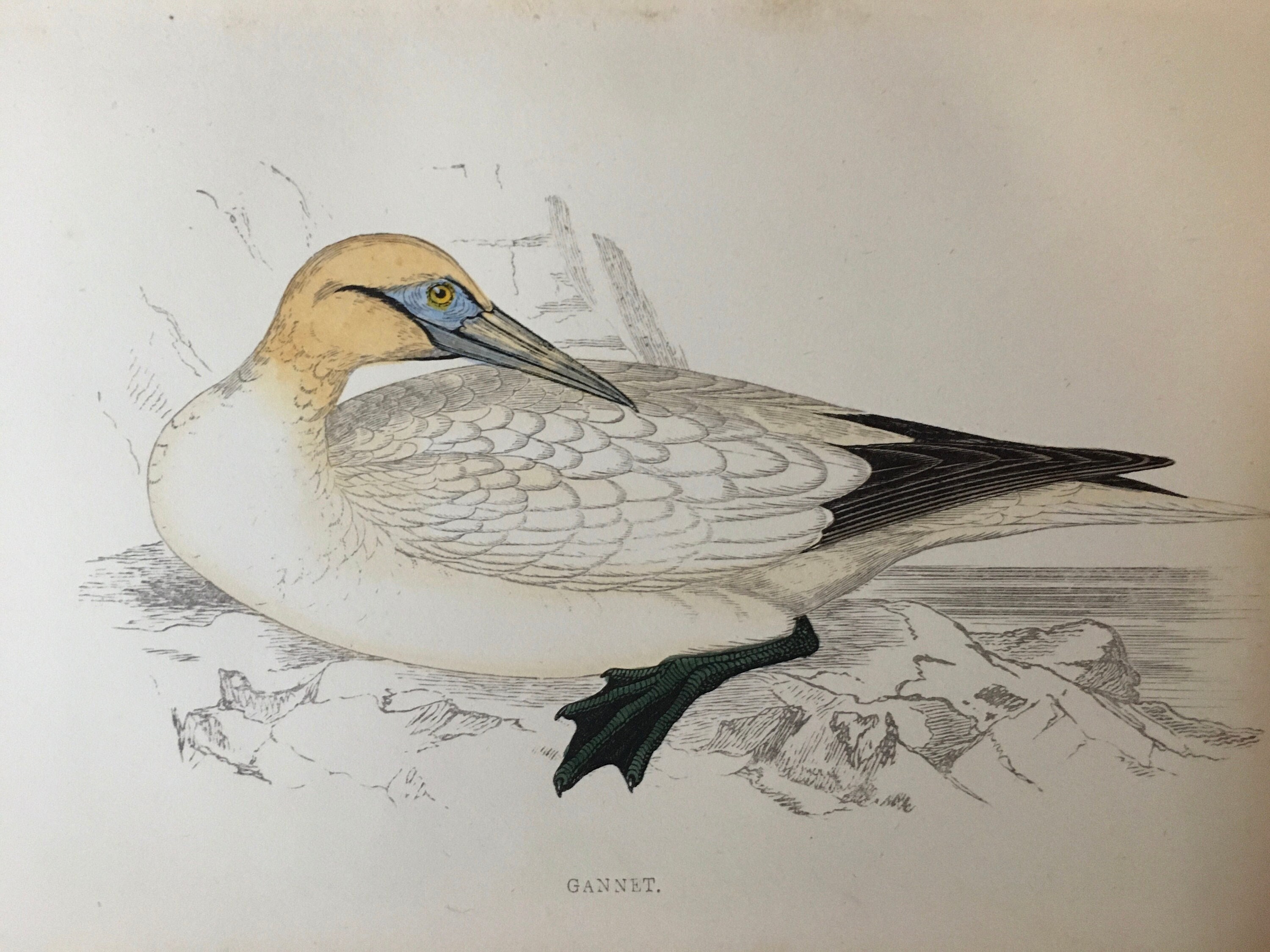This detailed illustration depicts a large, duck-like bird, reminiscent of Japanese art style, prominently positioned on a rocky ledge near water. The scene is rendered primarily in charcoal and pencil strokes. The bird, central to the image, is drawn with meticulous attention to detail, displaying a rich mixture of colors and textures. It features a yellowish beige head with a distinctive blue patch behind a yellow eye, and a long, striped beak. The bird's feathers are finely penciled, giving it an overall beige-white appearance, except for the black-tipped tail feathers which form a distinct triangular shape. Its body faces left, but the head is dramatically turned to the right, presenting its left-side profile with black and green webbed feet that show intricate ridges. Horizontal strokes in the background suggest a water setting. At the bottom of the image, the word "Gannet" is inscribed, crediting the artist or possibly the bird's species.